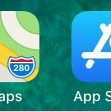This image is a small, approximately 1.5-inch square segment, extracted from a cell phone screenshot. The background is a rich and dynamic green, featuring various shades and textures to give the illusion of movement. This includes dark, almost black lines, some grass-like green areas, and lighter regions tinged with white. The image is filled with vibrant elements, including two prominent app icons. One is the Maps app icon, characterized by a tan background with a tan road cutting through it, patches of green representing grass, a yellow highway, and a blue route sign topped with red that reads "A to B." Adjacent to it is the App Store icon, which stands out with its blue background and a white "A" symbol at its center. All these details contribute to a visually engaging and textured appearance.